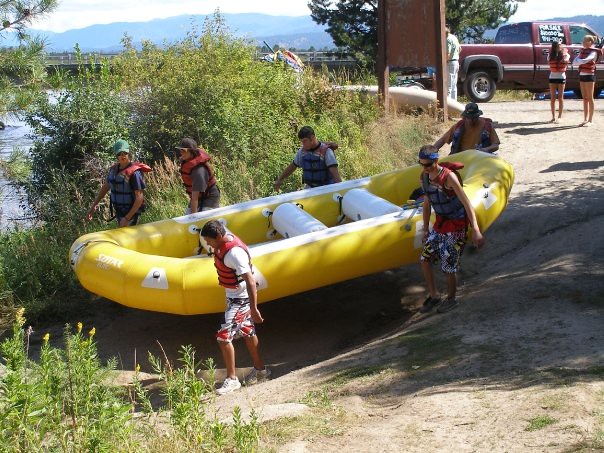In this photograph, six young men, likely in their teens or twenties, are carrying a large yellow and white rubber raft down an embankment towards the river's edge. Each of them is outfitted in colorful swimwear, t-shirts, and life vests, holding onto the raft, which features three benches across its center. The setting is vibrant with greenery, as weeds, little trees, and foliage fringe the river. 

In the background, the sun shines brightly despite a bit of haze over the mountainous horizon. 

To the right, two young women in shorts, t-shirts, and life jackets stand on a paved surface near a red pickup truck marked with 'for sale' and a phone number. Additional figures mill about at the top of the hill, where a rail—possibly a bridge or the water's edge—is visible. The scene is lively and brimming with anticipation as the group prepares for a rafting adventure.